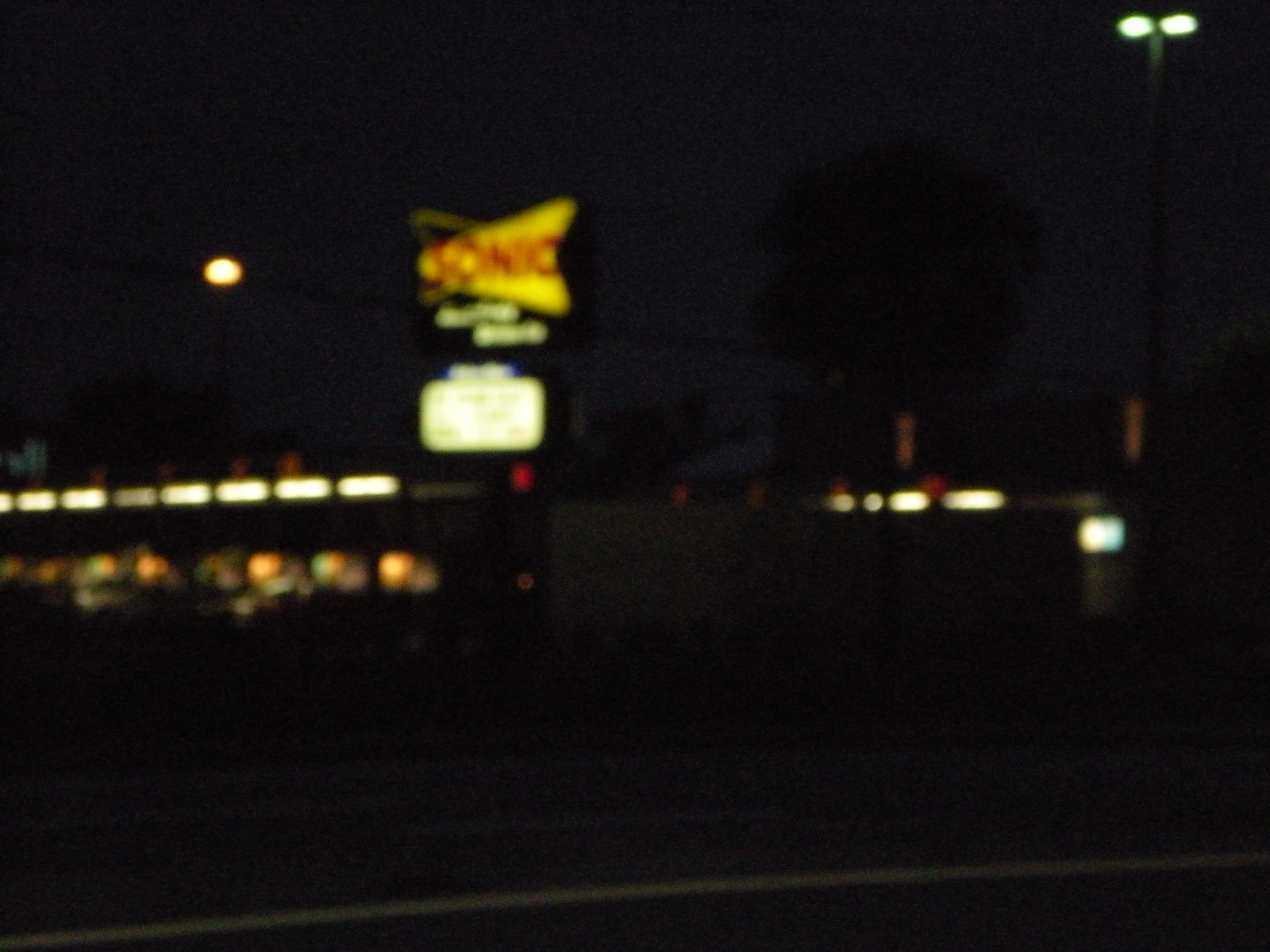The image captures a night scene outside a Sonic Drive-In restaurant. Dominating the scene is an illuminated sign displaying Sonic’s distinctive yellow logo against red lighting. Below the logo, there is some indecipherable white text. Beneath this text, a white illuminated sign is visible, designed for arranging letters into messages, though the current arrangement is unreadable. In the background, a building is outlined by a row of wide, short windows near its top, presumably the Sonic establishment. The faint glow beneath these windows hints at the border of a parking lot, with what seem to be a few indistinct, blurry cars. The surrounding area is enveloped in darkness, with a faint line at the bottom indicating the edge of a road. On the right side of the image, a tall pole with dual streetlights is visible, casting some light onto the scene. Additionally, a dim light floats in the air to the left of the pole, likely attached to another unseen pole.